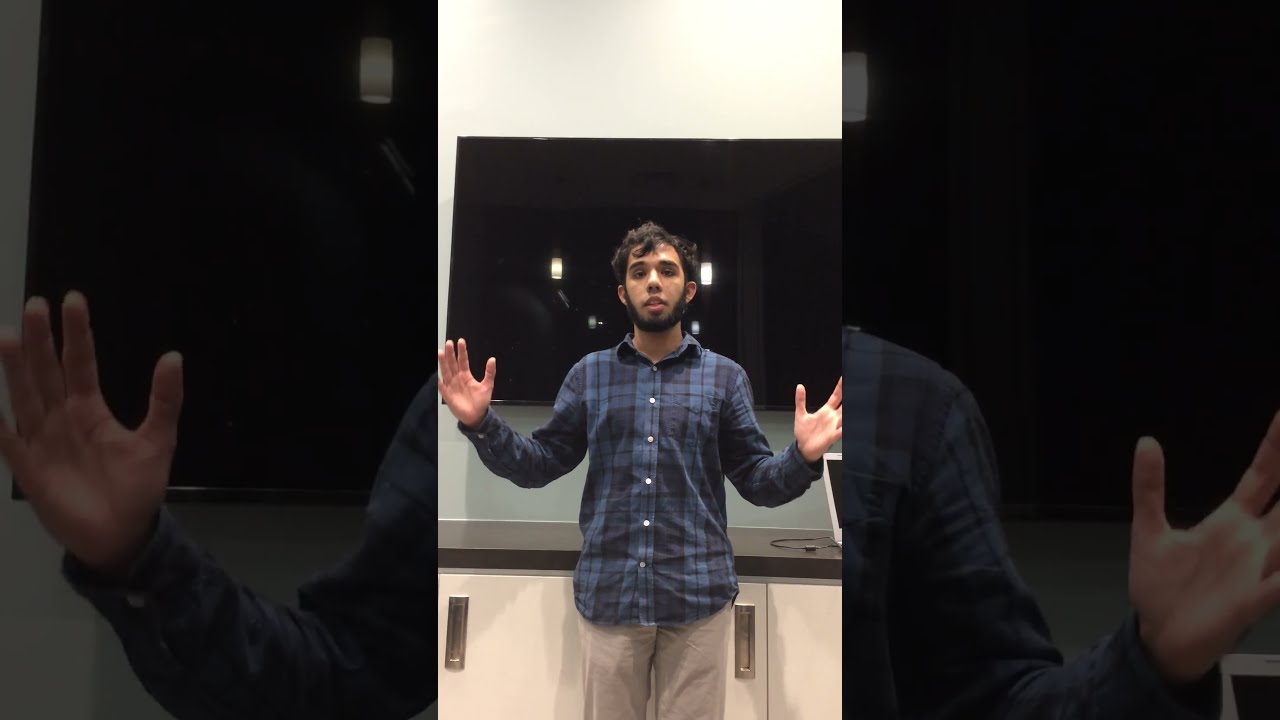This horizontally aligned rectangular image features a man facing the camera, centered within thick black borders on both sides, giving the impression of a vertically oriented rectangular picture in the middle. The man, with curly black hair and a dark beard but no mustache, dons a blue-black plaid long-sleeve button-down shirt. His hands are clasped in front of his chest with fingertips touching, suggesting a moment of conversation as his mouth appears open. 

He stands in front of a black TV screen that captures the reflection of lights from the room. The black, off-screen is mounted on a light-colored wall and below it is a brown countertop with cream-colored cabinets featuring brown handles. To the far right of the image, the edge of a laptop with a white border and a cord are visible against the counter. Additionally, the man seems to be wearing very pale khaki shorts. His eyes are directed downward, deep in thought or speech.